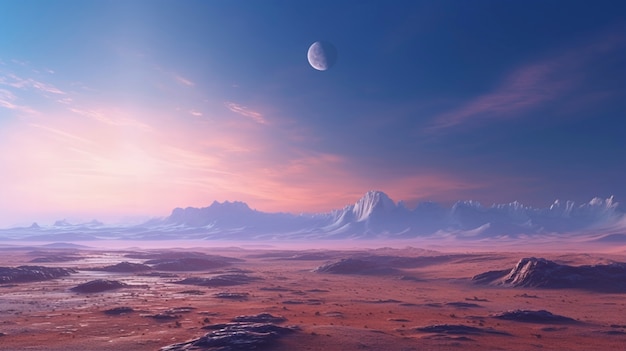The image, set outside, presents a surreal landscape that evokes a computer-generated or fantasy theme, resembling the surface of Mars. The terrain in the foreground is craggy, rocky, and of a rust and terracotta hue, typical of Martian depictions. The ground is dry and arid, with occasional rock outcroppings and mounds scattered throughout the dusty, clay-colored surface. 

In the distance, a rugged mountain range with various peaks stretches across the horizon. Above the mountains, the expansive sky transitions from deep blue to pink and white clouds, indicating a sunrise or sunset, with the sun positioned on the left side. Dominating the sky is a halfway illuminated moon, appearing faint as it would in the daytime, centrally placed amidst the colorful expanse. The combination of the surreal terrain, dramatic skies, and celestial bodies renders a strikingly otherworldly scene.